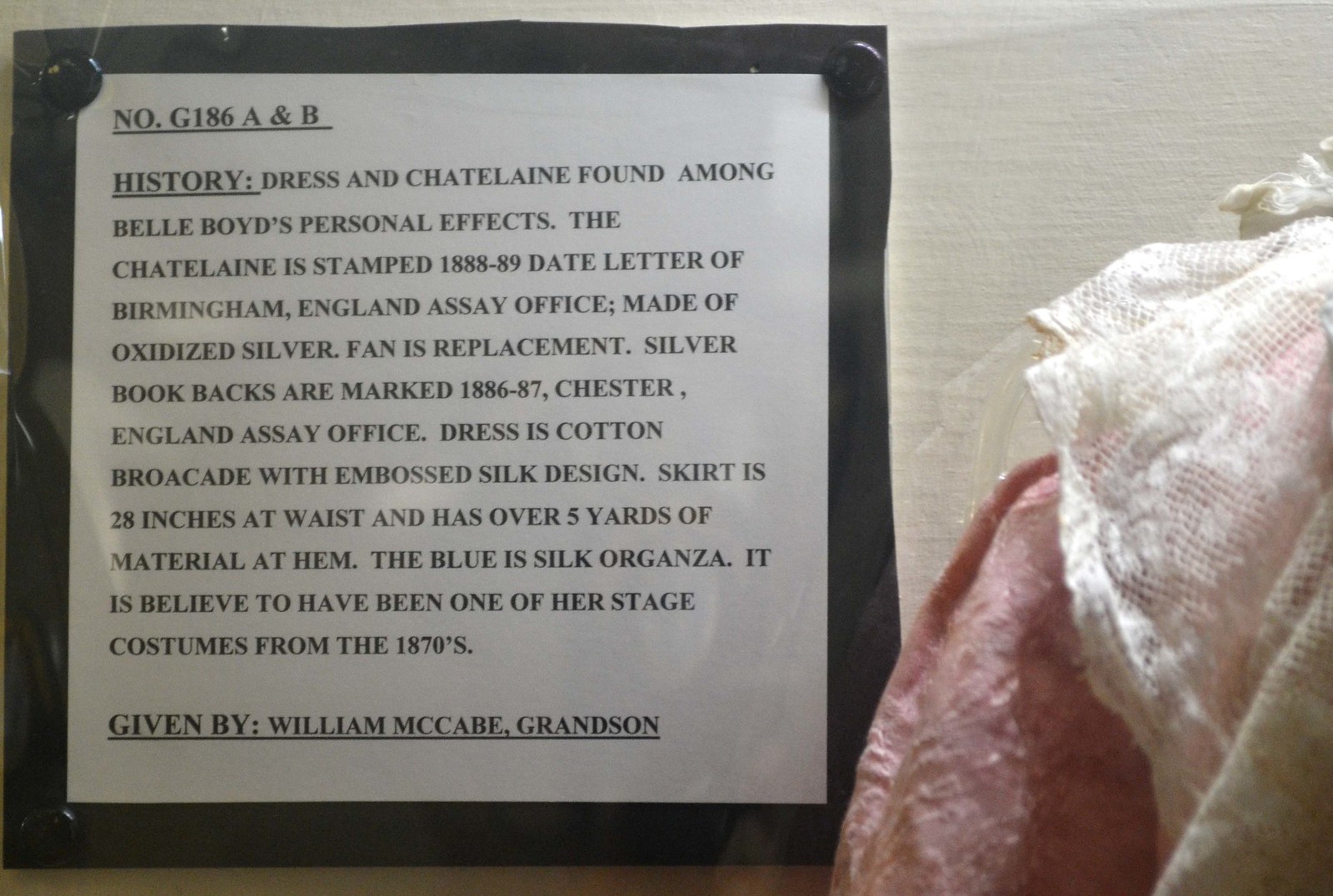This image features an informational sign displayed against a white wall, bordered in black with black thumbtacks securing it at each corner. The sign, written in black text on a white background, reads Number G186 A and B. The heading, "History," introduces the exhibit: "Dress and Chatelaine found among Bella Boyd's personal effects." The Chatelaine is noted to be stamped with the date 1888-89, from the Assay Office in Birmingham, England, and is made of oxidized silver. A note states that the fan is a replacement. Additionally, silver book backs are marked 1886-87, from the Assay Office in Chester, England. The dress is described as cotton brocade with an embossed silk design, featuring a skirt that measures 28 inches at the waist and contains over 5 yards of material at the hem, the blue elements being made of silk organza. It is believed this dress was one of Bella Boyd's stage costumes from the 1870s. The exhibit was a donation from her grandson, William McCabe. To the right of the sign, a small portion of pink and white fabric, including brocade and lace, is visible, likely part of the dress described.